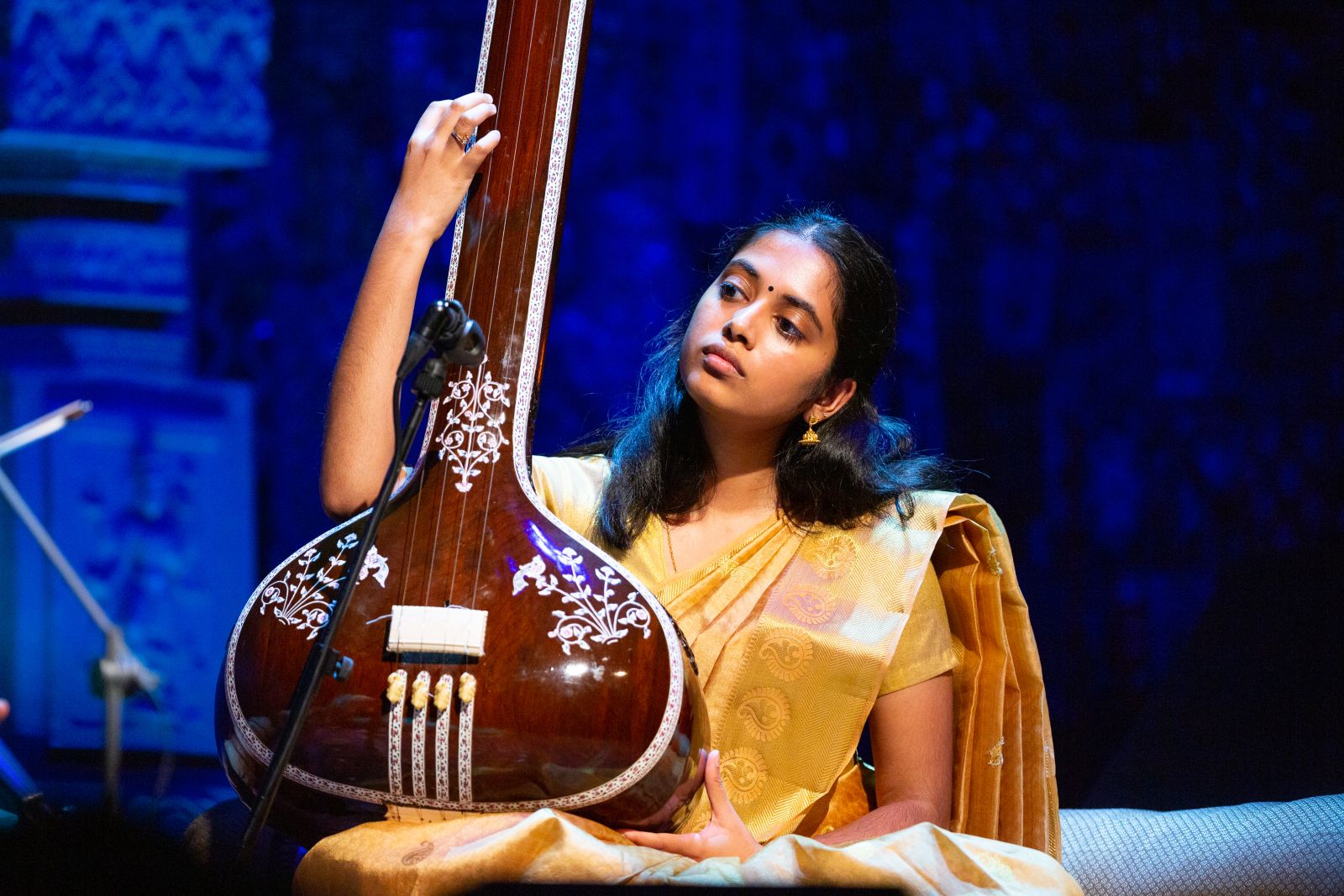The image is a realistic, horizontally oriented photograph, capturing a scene set against a blue-toned stage background with blurred decorations. Central to the foreground is a woman of Asian-Indian descent, appearing to be in her late teens to 30s, characterized by her black hair, light brown skin, and a decorative dot between her eyes. She is adorned in a yellow sari or robe made of ornate, thick fabric adorned with a small embellishment. She is seated, with a dark brown, highly ornate stringed instrument on her lap, resembling a sitar, featuring white decorations and floral shapes. Her right hand is wrapped around the neck of the instrument, touching one of the four strings, while a boom microphone is positioned nearby, directed towards the instrument. She wears gold earrings, has a ring on one of her fingers, and gazes attentively at the instrument, all under bright studio lighting that reflects off the medium chestnut brown wood of the instrument.